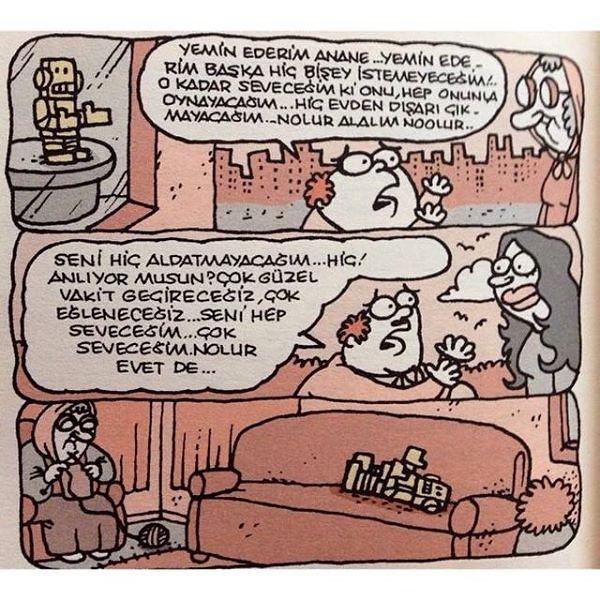The image is a scan of a three-panel comic strip with a tan background and black wavy outlines around each panel. In the first panel, a small robot sits on a gray pedestal in the upper left corner, with a tan-colored skyscraper visible in the background. A red-haired boy with big, sad eyes is talking animatedly in a foreign language to an older woman with glasses and a shawl over her head. In the second panel, the same boy, now older and sporting a mustache, continues to speak in the same foreign language, but this time to a younger woman with long black hair. The third panel showcases the older woman from the first panel seated in a chair to the left, knitting with a ball of yarn on the floor next to her. On an orange couch to the right, the small robot from the first panel is lying on its back, staring at the ceiling. The overall aesthetic of the comic appears to be vintage, rendered in a palette of tan, gray, orange, and black.